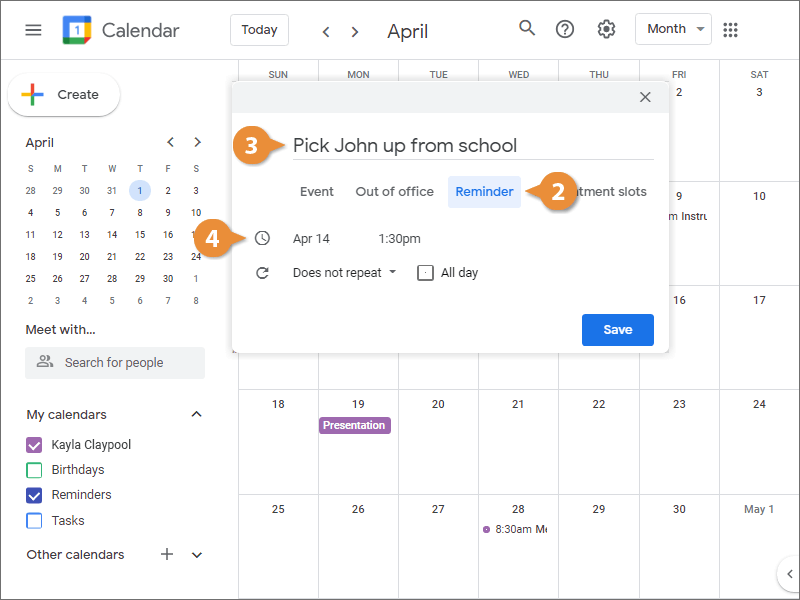This is a detailed photo of a calendar app, captured in a square format with a thin black border framing the image. The calendar is set against a pristine white background. At the top, there is a narrow gray border featuring several functional icons: a hamburger menu, a calendar icon with the familiar blue, yellow, red, and green Google colors, and the word "Calendar" beside it. This section also includes a gray "Today" button, flanked by backward and forward arrows, with the word "April" indicating the current month. A search bar, a question mark for help, a settings icon, and a drop-down box with "Month" selected are also visible in this section.

On the left side, in a small font, the sidebar displays the mini version of the calendar with all the dates. The main calendar occupies the center of the image, displaying a detailed layout of the month of April. Notably, a rectangular pop-up listing at the top has a thin gray border and the header that reads "Pick Sean Up from School." Adjacent to this, an orange text bubble with the number "3" points to this event. Below it, another orange text bubble labeled "4" pointed to a clock icon. A light blue reminder box with dark blue text is marked by a "2" text bubble placed next to it. Other entries such as "Presentation 8:30 AM" and "Meeting" are marked on the calendar, providing a detailed overview of scheduled events and reminders for the month.